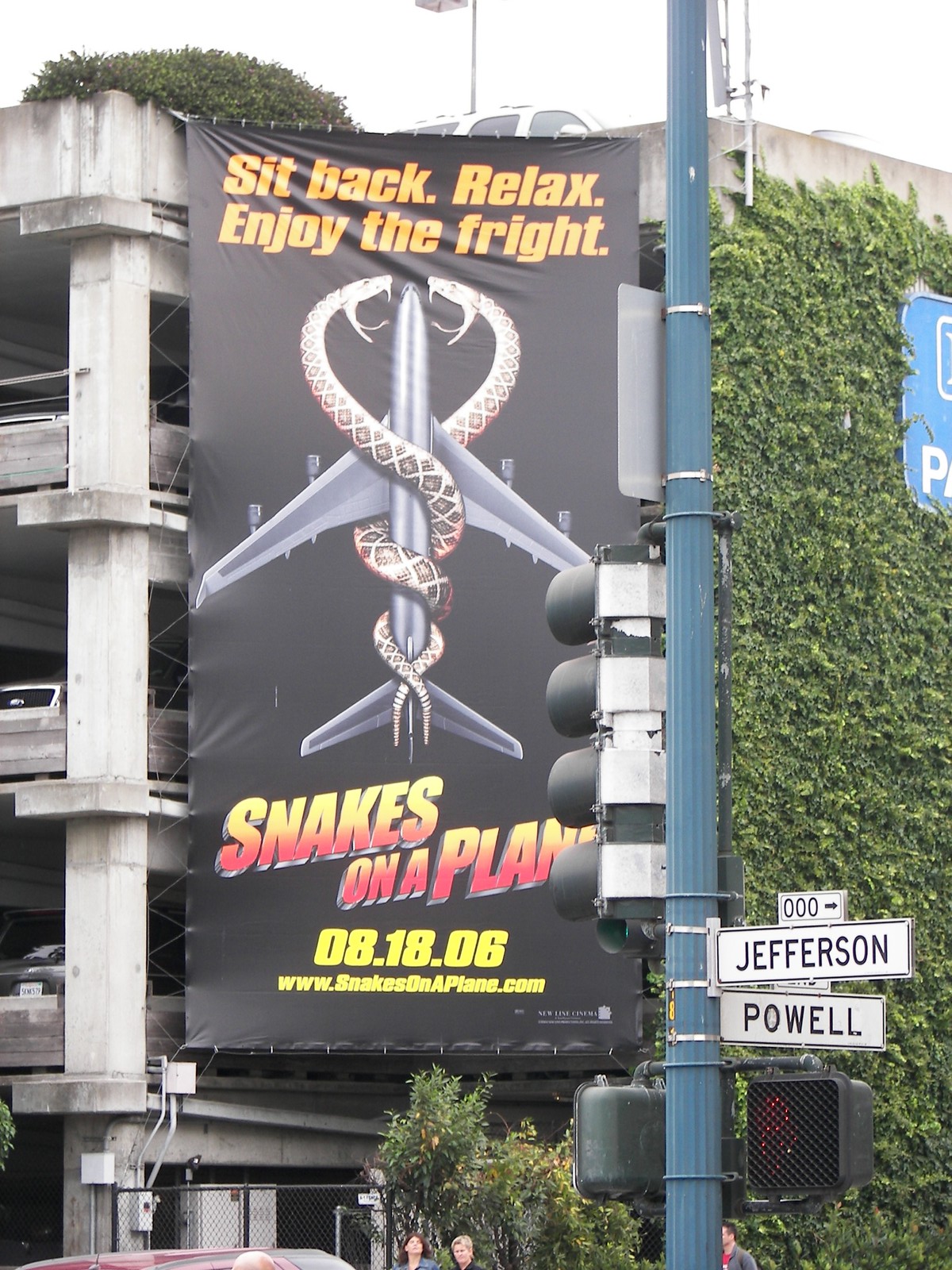The image depicts an advertisement poster mounted on the side of a parking garage situated at a street corner. The prominent feature in the foreground is a dark teal-colored street lamp fitted with street signs labeled "Jefferson" and "Powell" in white with black lettering. Below the street lamp are black boxes housing the walk and stop crosswalk signals and a traffic light. The background features the parking garage, with its right side densely covered in green ivy. The left side of the garage showcases exposed gray concrete and the tops of several parked cars. The large banner on the garage wall is an advertisement for the movie "Snakes on a Plane," prominently featuring the film's logo, a movie description, and its tagline.